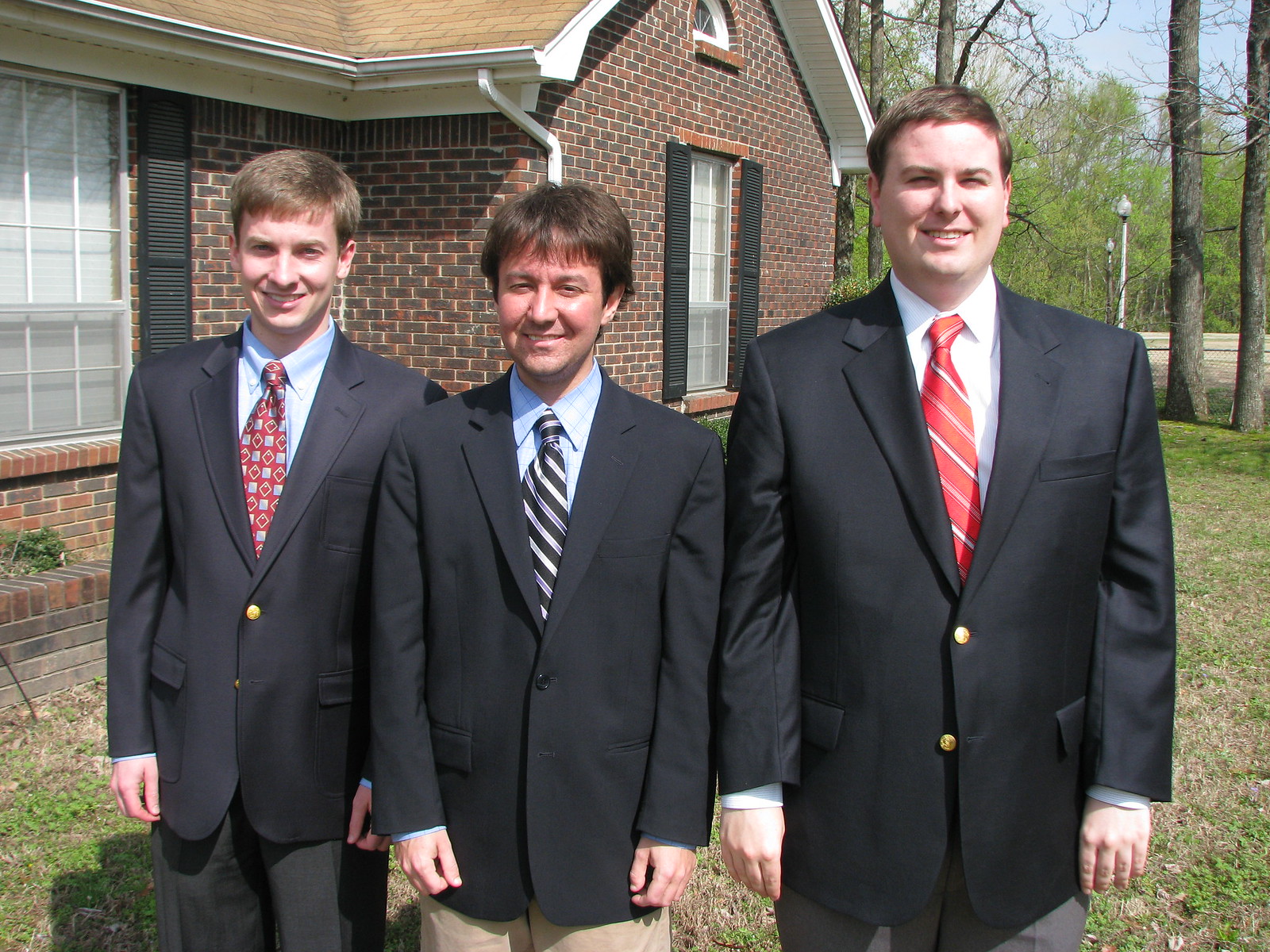In this detailed, landscape-oriented image, three young men, who could be older teenage boys, stand side by side, smiling at the camera on a clear and sunny day. All three are dressed in black suits with neatly buttoned jackets, white collared shirts, and ties, each varying in pattern and color. The man on the left sports a red patterned tie paired with grey trousers, and the man in the middle wears a black, blue, and white striped tie with beige trousers. The man on the right, slightly bigger and younger, dons a red and white striped tie with light grey trousers. They all have short brown hair and stand with their hands resting by their sides. Behind them stands a brick house, brown and red in color, with large windows. The scene is complemented by a few tall, brown trees with twigs and patches of greenery, hinting at an early spring or late fall setting. A streetlight can also be seen, adding to the suburban backdrop.